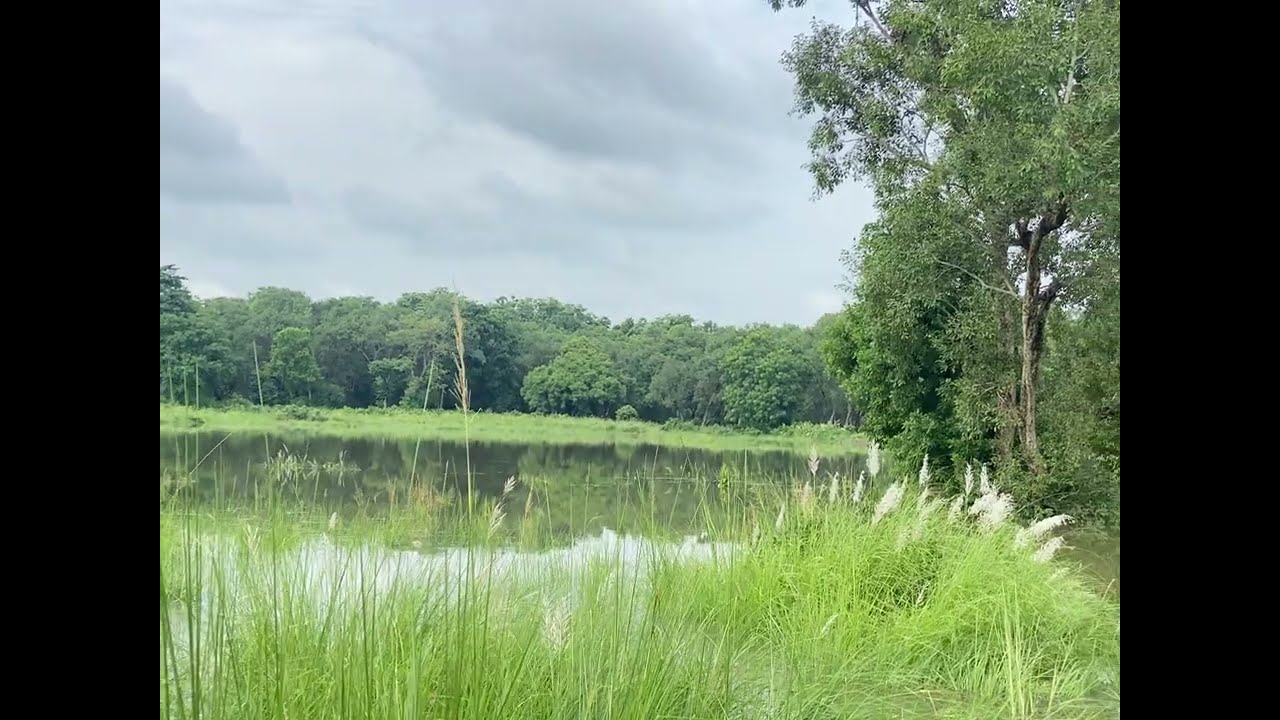This detailed landscape photograph captures a tranquil marshland scene on an overcast day. In the foreground, ample tufts of sawgrass, with stalks reaching up to four feet tall, dominate the lower portion of the image. Just beyond these grasses, a serene pond or lake stretches into the distance, its smooth, reflective surface mirroring the surrounding vegetation. The water is pristine, contributing to the overall clean and calm atmosphere of the environment. On the right side of the scene, a portion of the near bank is visible, characterized by robust, green vegetation. The far bank, approximately two to three hundred meters away, is a verdant expanse lined with an array of dense, tall trees, suggesting the edge of a thick forest. The sky above appears cloudy, covering about half of the image and lending a muted light to the landscape. Overall, the image evokes a sense of stillness and untouched nature, absent of any human presence or text.